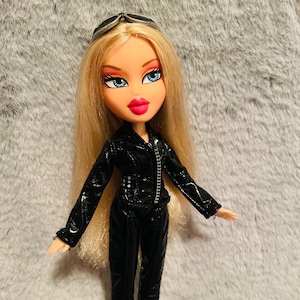The image depicts a small square photograph of a doll that closely resembles a Barbie but stands out due to its distinctive features. The doll, with a disproportionately large head for its slender body, has long, straight, blonde hair extending down to the back of its thighs. She sports perfectly curved brown eyebrows, large blue eyes with pronounced eyelashes, and dark red lipstick on her prominent, animated lips, giving her a striking and almost exaggerated appearance. Her outfit consists of a long-sleeved black top with a zippered front adorned with a white pattern, paired with black leather pants. Sunglasses with a brownish bronze frame and black lenses rest atop her head. The doll is set against a textured, cream-colored, fuzzy background, casting a shadow that suggests a light source from the top right. She is positioned with her arms slightly raised from her sides and her gaze directed towards the right side of the photo, contributing to her poised, yet blank expression.